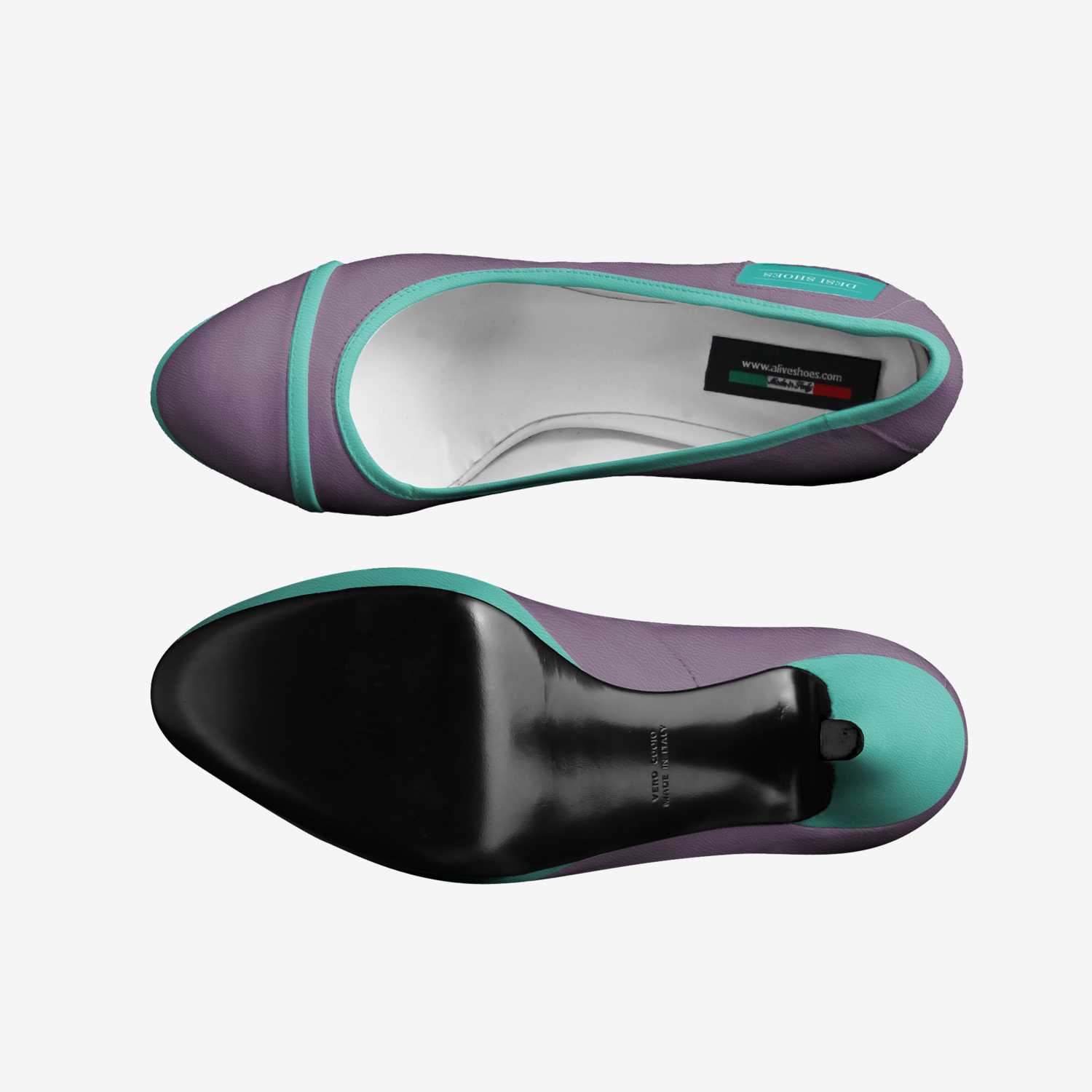The image showcases a pair of women's flats in an overhead view, set against a plain white background. The shoe on the top displays the upper part, revealing a purple exterior with a turquoise blue trim around the opening where the foot slides in, as well as a turquoise band near the toe. The inside of this shoe is silver and contains a tag from the brand AliveHues.com. A smaller tag inside the shoe features green, white, and red colors, reminiscent of Italian or Mexican style. The shoe at the bottom shows the underside, which has a black rubber or leather-style sole, complemented by turquoise trim near the upper part. Both shoes are aligned with their toes pointing to the left and heels to the right, with a blue tag visible on the back of the right shoe for added detail. The overall design highlights a looping, curvature shape for comfort both inside and outside the shoes.